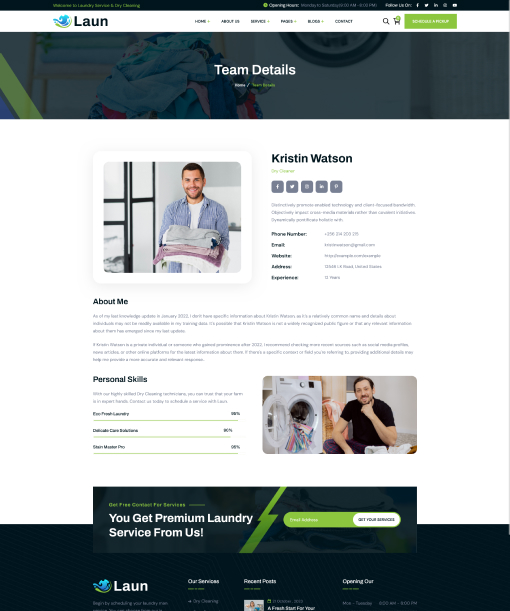In this image, we see the homepage of a website created by LAUN, with the brand name "LAUN" prominently displayed in black letters at the top-left corner. To the right of the brand name, there are several small clickable options, though their specific functions are not readable in this image. Adjacent to these options is a rectangular search bar accompanied by a search icon.

The main section of the website features a large dark blue rectangle with the text "Team Details" written in white. Below this header, there is a photograph of a man named Kristen Watson holding laundry. His contact information, including phone number and address, is listed beneath his picture alongside a section labeled "About Me." Another image of Kristen next to a washing machine and dryer accompanies this section, highlighting his personal skills.

Further down, the text reads, "You get premium laundry service from us," indicating that this website is a career services platform offering professional laundry services. Kristen Watson appears to be a service provider who offers laundry services, potentially for both individual and corporate clients.